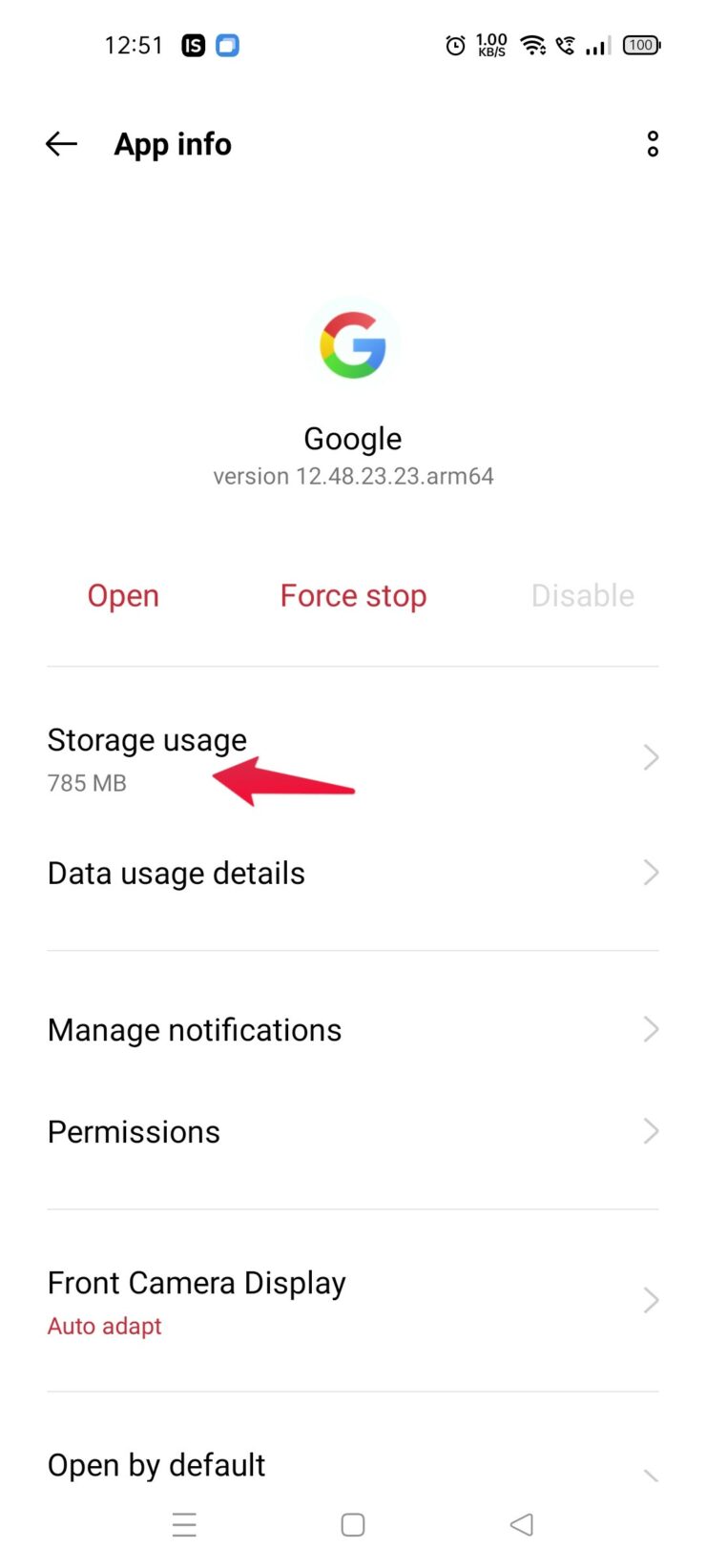The image is a detailed screenshot of the app information page for the Google app on a mobile device.

At the very top of the screenshot, the current time is displayed as 12:51. To the left of the time, there's a black oval icon with the letters "IS" in white. Just to the right of that, there's a blue oval with a plain white center. Further to the right, there is an alarm clock icon, followed by another icon marked "1.00 KB/s". Adjacent are various status icons including a Wi-Fi symbol, a phone with a Wi-Fi calling icon, a signal strength indicator showing three black bars and one gray bar, and a battery icon indicating 100% battery life with two small black circles beneath it.

Below the time on the left side, there is a left-facing arrow labeled "App info" in black text. Centrally positioned, the multicolored "G" Google logo is displayed (red, yellow, green, blue). Beneath the logo, the word "Google" is spelled out in black text with the version number "12.48.23.23.ARM64" rendered in gray below.

Moving down, there are three buttons: "Open" in red on the left, "Force Stop" in the center, and "Disable" which is grayed-out on the right. A light gray line demarcates this section from the subsequent details.

Below this line, on the left side, "Storage usage" is written in black text with a thick red arrow pointing towards the value "75 MB" in gray. On the right, there is a right-facing triangle icon. Subsequent sections are listed in black text, each separated by light gray lines and featuring right-facing triangle icons: "Data usage details", "Manage notifications", "Permissions", followed by "Front camera display".

The next item, "Auto-adapt," is highlighted in brown text, accompanied by a gray line and a right-facing arrow. Finally, "Open by default" is listed. 

At the bottom are symbols commonly found on cell phones: three horizontal lines, a square, and a left-facing arrow, all summing up the detailed and informative screenshot.